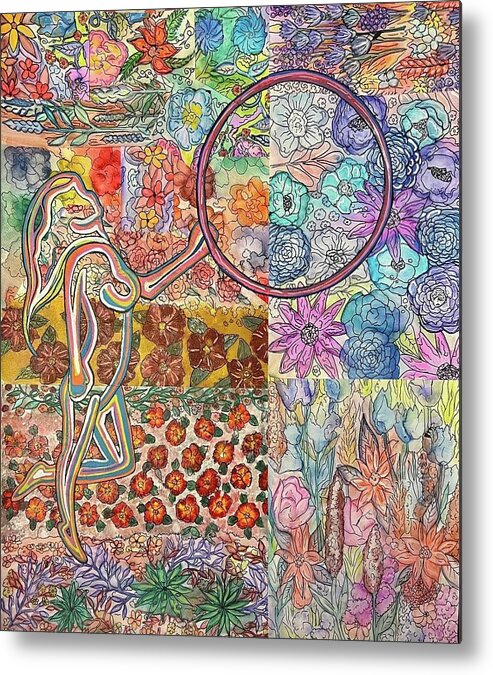This vivid and intricately detailed painting exudes the charm of an adult coloring book, meticulously sectioned into various panels featuring a captivating array of flowers. Each panel bursts with its own unique color palette, ranging from sets of turquoise, blue, and purple blossoms, to clusters of vibrant yellow, dark red, and green florals, and swathes of orange, purple, and yellow blooms. The floral designs often intertwine, creating a cohesive yet diverse tapestry of hand-colored petals that cover every inch of the canvas.

On the left side of the image, a stylized and ethereal outline of a woman emerges. This figure, with long, flowing hair and a serene expression, appears to levitate gracefully. She holds a large, red hoop in her left hand, further accentuating her floating form. Her pose is both elegant and dynamic, adding an expressive, almost magical element to the already mesmerizing composition of the painting.